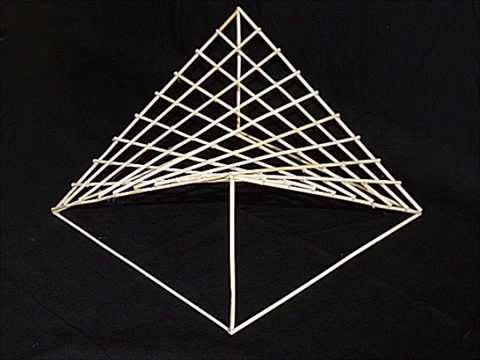The image depicts an intricate, geometrical structure resembling a skeletal kite set against a stark black background. Dominantly white and composed of twig-like sticks, the figure features a prominent diamond shape forming its perimeter. The upper portion of the structure is filled with an elaborate, crisscross pattern of smaller rhombus-like diamonds, creating a complex and almost three-dimensional perspective that hints at a triangular prism upon initial inspection. However, closer examination reveals the bottom portion to be empty of such patterns, revealing a base that appears to be a square split diagonally. Overall, the composition blends elements of forced perspective and geometric abstraction, making the image both visually puzzling and intriguing.